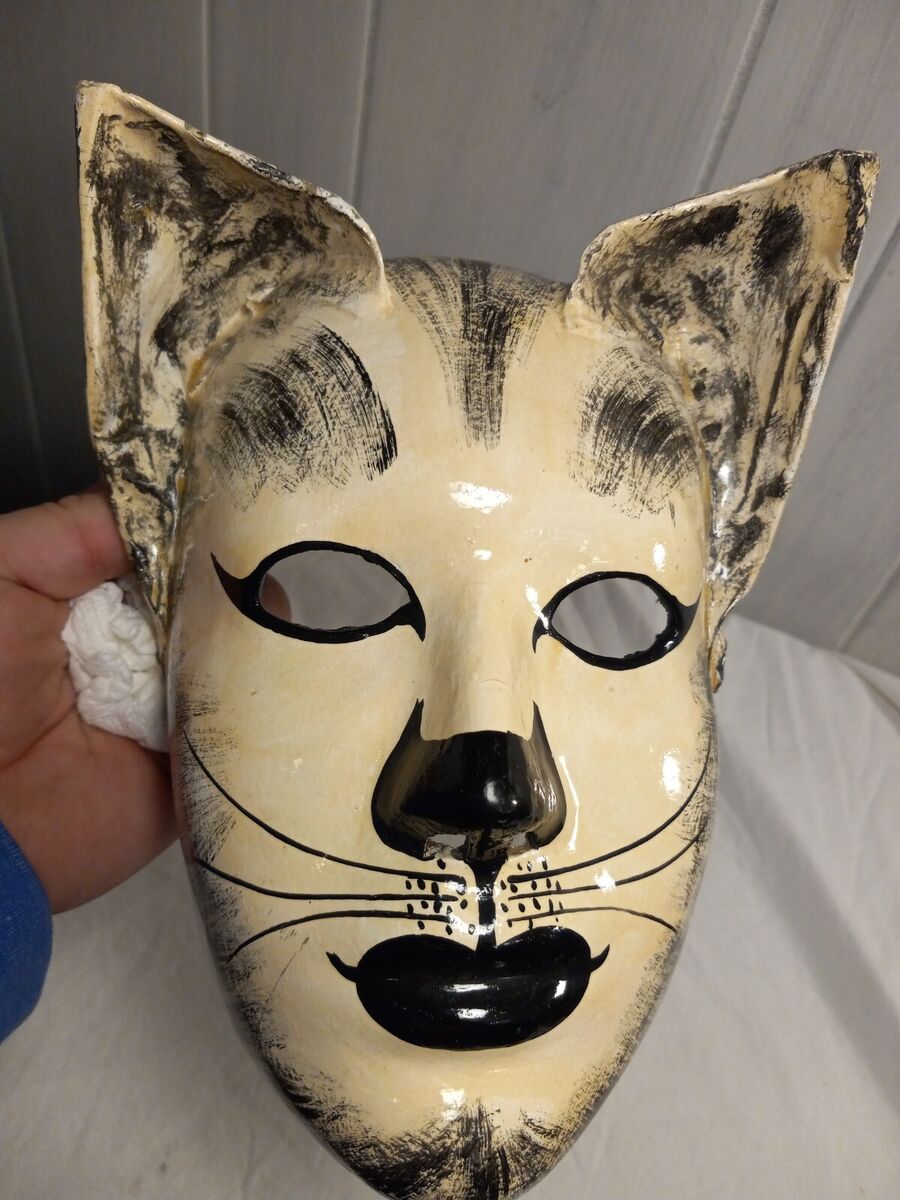The image features a detailed, glossy, paper mache-style cat mask centrally positioned against a two-tone background. The cat mask, sophisticated and possibly used in performances, exhibits beige hues with intricate black detailing: dark, prominent cat eyes, a black nose, whiskers emanating from dots near the nose, black lips, and black fur-like stripes framing the face and extending from the eyebrows towards the edges. The mask also has distinctive, pointy ears. A hand, holding a tissue for careful handling, is located to the middle left, highlighting the mask's delicate, possibly glass-like nature. The background comprises a textured white wooden wall on the upper half and a soft, fabric-like material, possibly a tablecloth or bedsheet, on the lower half, suggesting a casual display setting. The mask’s significant presence dominates the photo, underscoring its likely value and fragility.